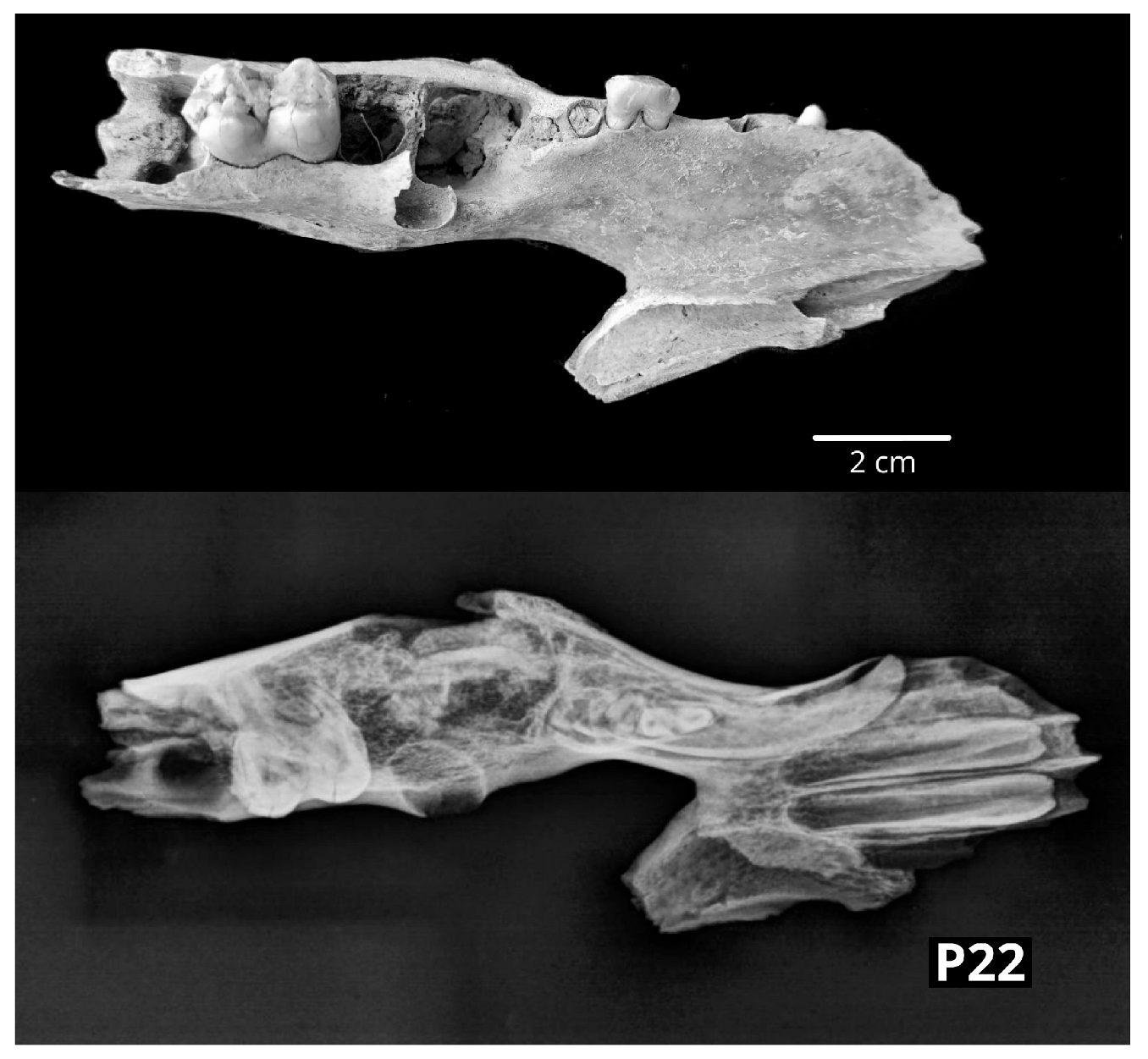The image comprises two black-and-white photographs of the same object, displayed one above the other. The top photograph shows a physical depiction of what appears to be an animal's jawbone, likely fossilized, complete with a few visible teeth. This image features a black background and includes a scale bar indicating 2 centimeters to provide a sense of size. The bottom photograph is an x-ray of the same jawbone, revealing more intricate internal structures that are not visible in the top photo. The x-ray background is slightly lighter, and it bears the label "P22" in white text on a black box in the bottom right corner. The teeth visible in the jawbone include some molars with distinct roots and some empty tooth sockets, suggesting this is part of a mandible from a larger animal, possibly prehistoric. Both images highlight different aspects of the jawbone, with the x-ray providing a translucent view that reveals cavities and internal details, enhancing the overall understanding of the fossil's structure.